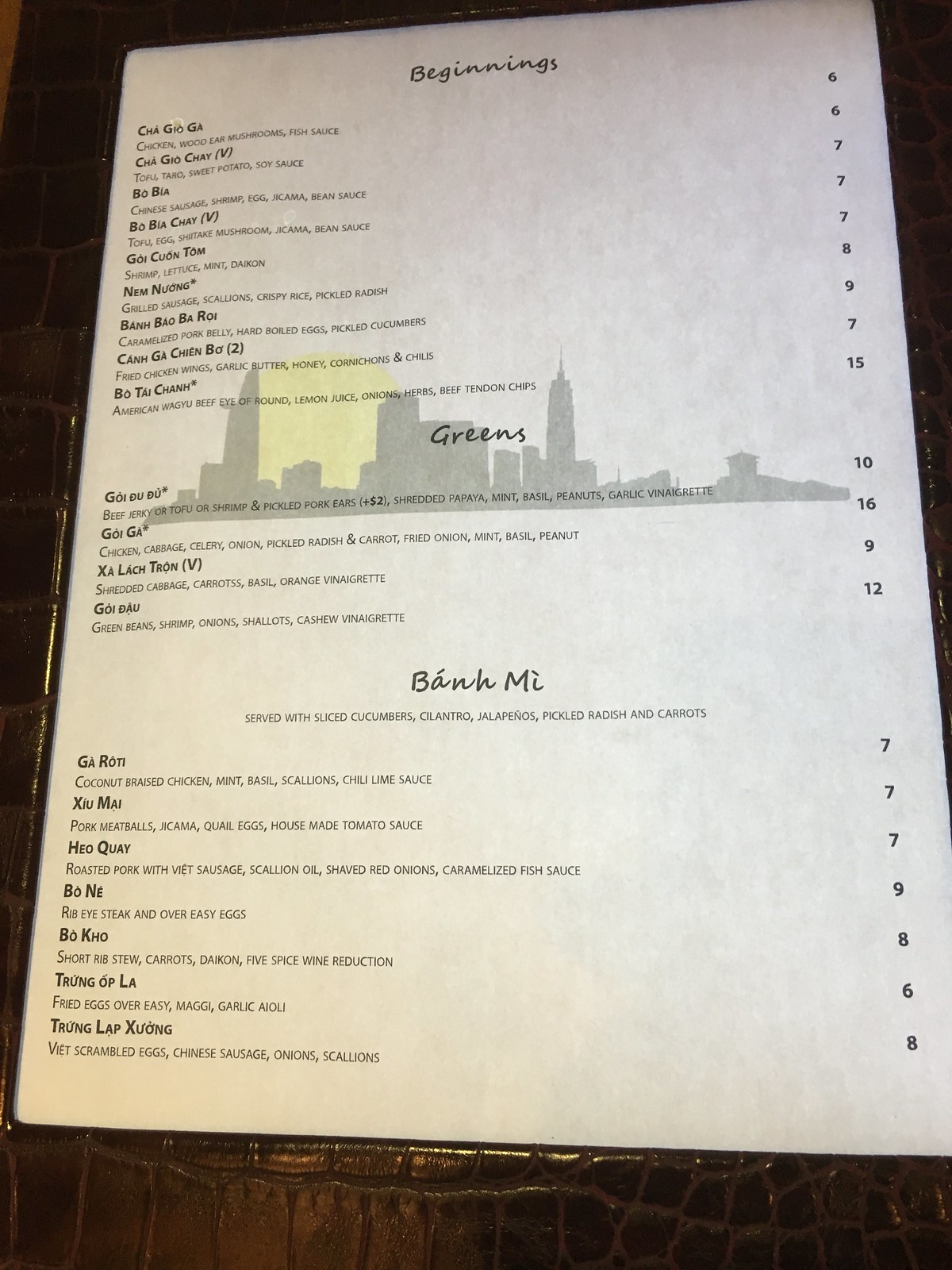This image captures a restaurant menu encased in a sophisticated faux alligator skin holder, designed with a plastic window for easy menu updates. The holder is likely bi-fold, providing a sturdy alternative to a mere paper sheet. The menu is elegantly categorized into three sections: Beginnings, Greens, and Banh Mi. On the left side, each dish is briefly described, while the corresponding prices are listed on the right. 

The Beginnings section features an assortment of appetizers, the Greens section offers various salads, and the Banh Mi section showcases a variety of Vietnamese sandwiches. A highlighted dish named "Gai Rati" consists of coconut-braised chicken garnished with mint, basil, scallions, lime, and chili sauce. All Banh Mi sandwiches are served with fresh sliced cucumber, cilantro, jalapenos, pickled radish, and carrots. This detailed menu offers a glimpse of the diverse and flavorful offerings at this Banh Mi restaurant.